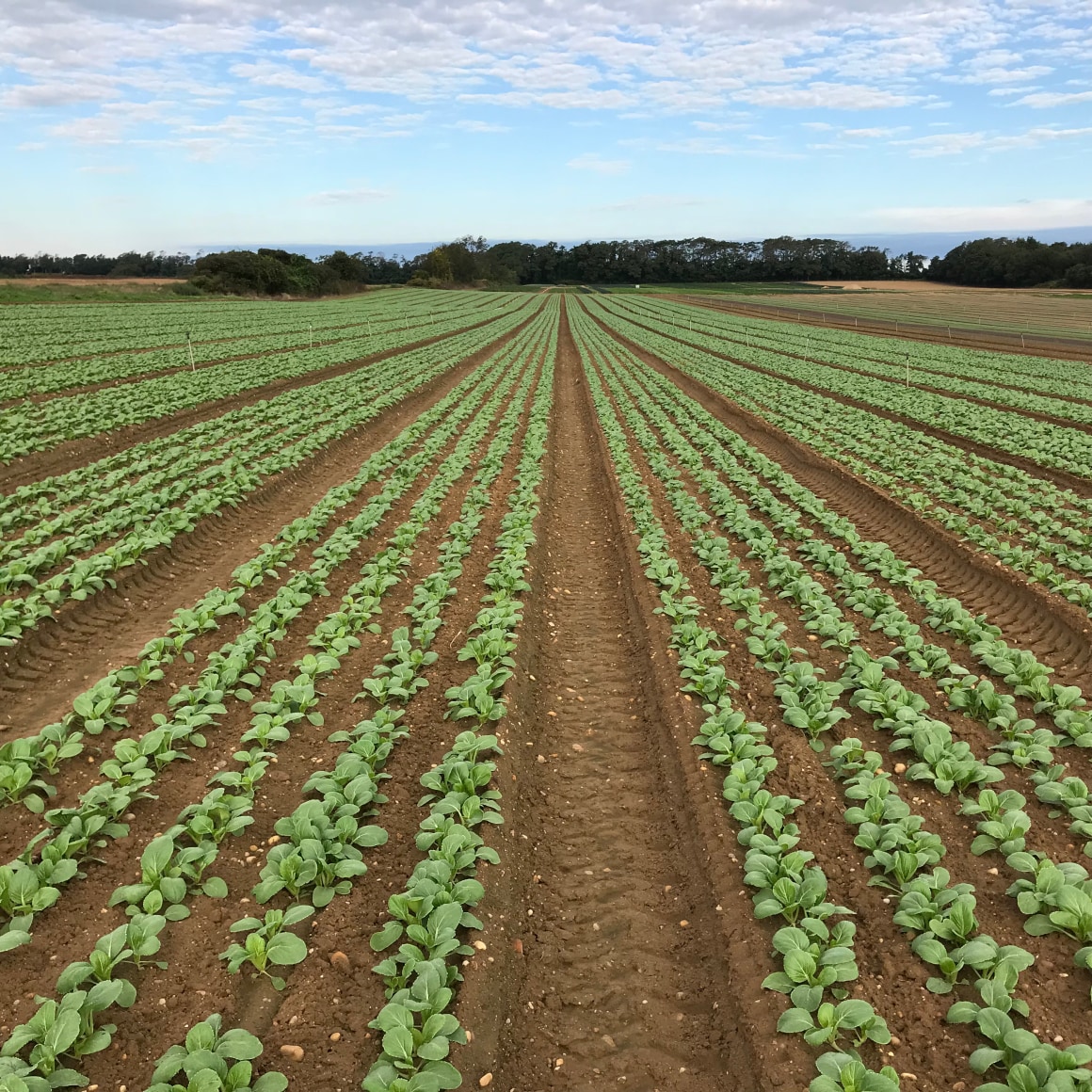The photograph depicts a vast farmland with meticulously arranged vertical rows of small, green leafy plants growing close to the ground, possibly a type of leafy vegetable. The soil appears light brown and somewhat rocky, interspersed with what looks like light yellow wood chips or shavings. Visible tire tracks, visible between every five rows, suggest recent tractor activity for irrigation. In the far distance, the horizon is lined with dark, large trees and possibly a small white building. Sprinklers are also noticeable on both the left and right sides of the field. The sky above is light blue, adorned with scattered clouds, adding to the picturesque landscape. The image is a vivid blend of cultivated land, structured agriculture, and natural background elements.